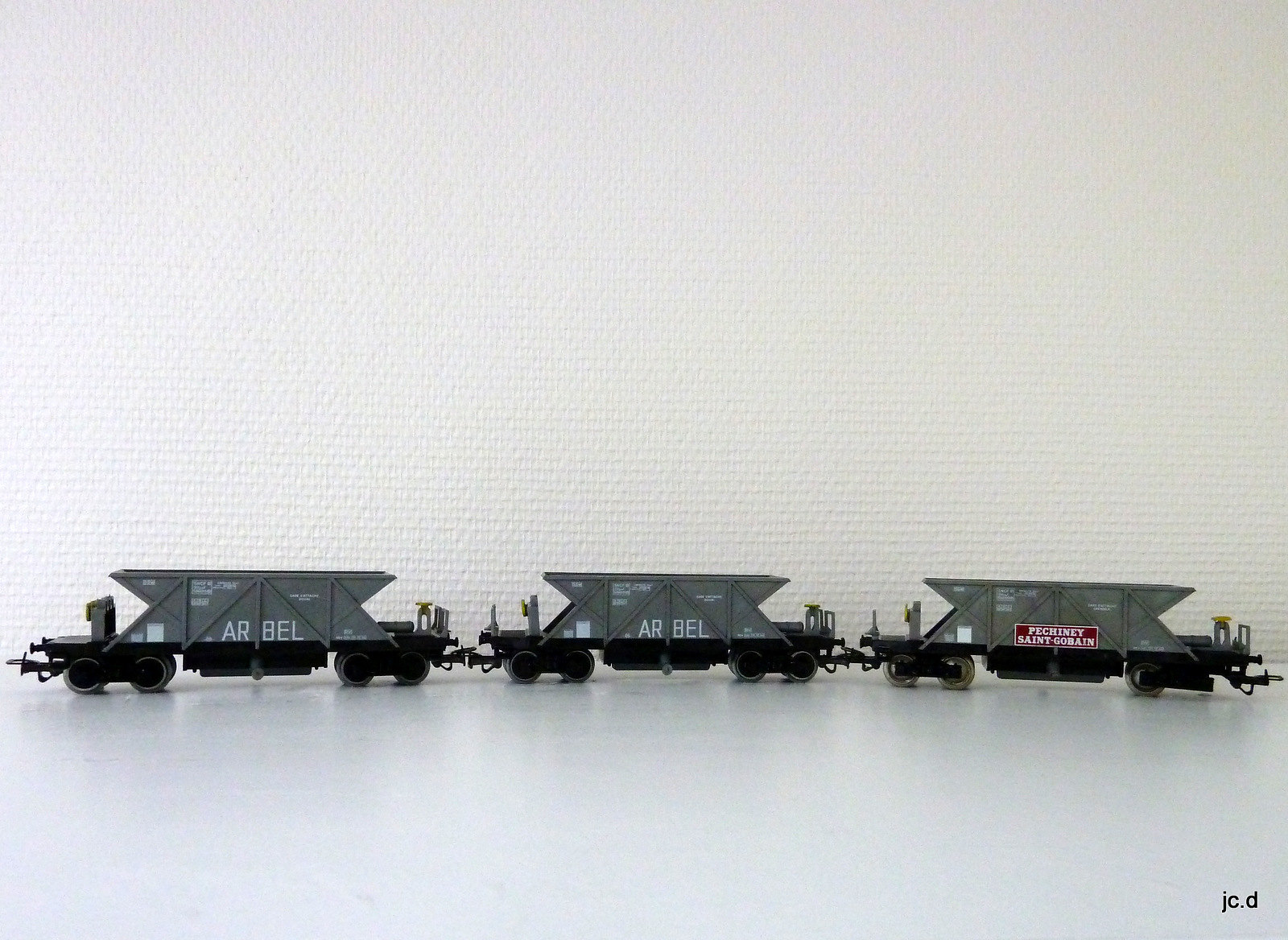This photograph showcases three toy train carriages, each meticulously designed with a rectangular shape featuring pointed ends. The carriages, which are dark grey in color, are mounted on black frames supported by sets of eight wheels. They are interconnected, forming a miniature train that runs from the right to the left across the bottom of the image. The toys are positioned on a white surface against a white wall with subtle vertical textures.

Each carriage has distinct markings: two of them display the letters "AR BEL" in white, while the third features a red and white label that reads "Pecheni Saint Gobain." Additionally, the bottom left corner of the image includes the initials "JC.D" written in black. The intricate details of the carriages and the precise arrangement against the stark background emphasize the craftsmanship of the miniature toys.